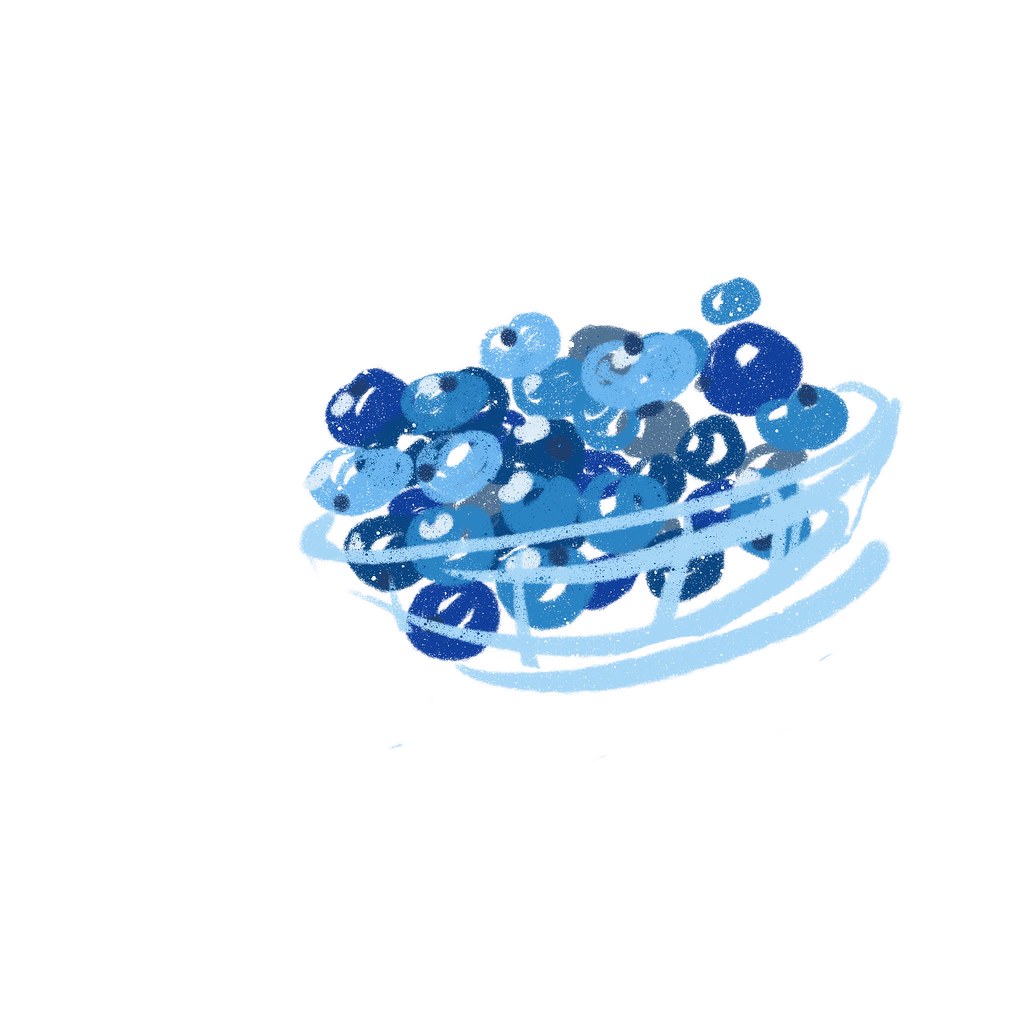This artwork features an abstract, clip art-style illustration of a light blue bowl, depicted with simple and translucent blue circular and vertical lines that give it the appearance of a straw or wire basket. The bowl holds an assortment of berries, primarily blueberries, in varied shades of blue, ranging from deep blue and periwinkle to lighter and grayish blue hues. The artist has added small blue dots as well as touches of white and black on the berries to create contrast and texture, making some berries appear almost dark gray or deep purple. The background is plain white, highlighting the predominantly blue color scheme and minimalist style of the painting.